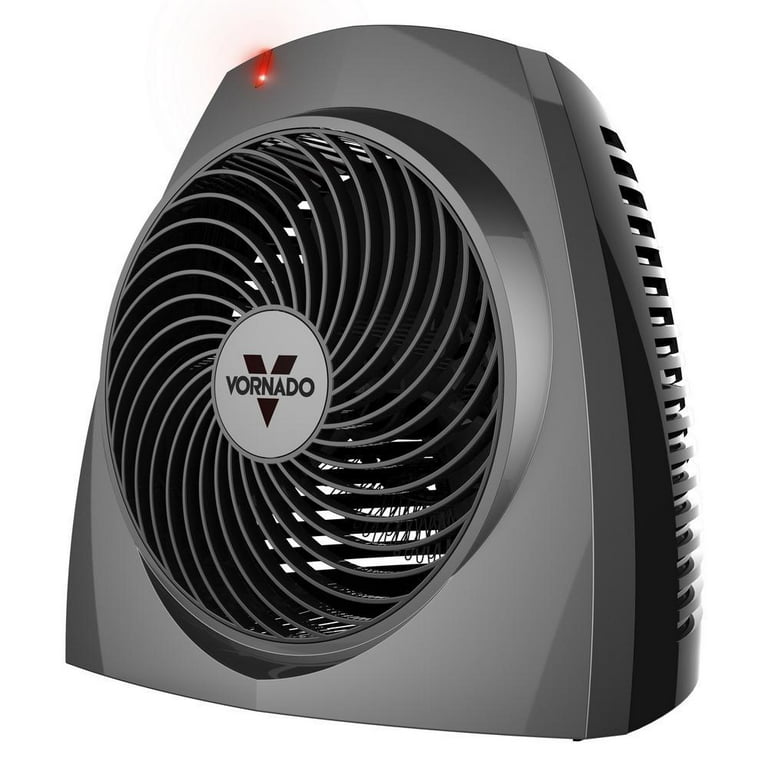The image depicts a small, black plastic tabletop fan with a flat base suitable for placing on a table or floor. The fan is branded Vornado and features a front circular vent with internal fan blades, highlighted in light gray. In the center of the vent, a prominent black capital "V" intersects with the brand name "VORNADO" displayed in black letters. The upper part of the fan is rounded with a red light indicating power status. The device is square-shaped overall, with rectangular openings and ridges on the back for ventilation. The background of the image is white, providing a clear contrast to the black and gray colors of the fan.